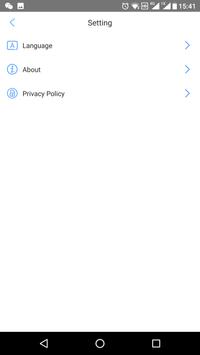The image appears to be a screenshot taken from a cell phone, displaying a settings menu. At the top, there is a gray horizontal bar extending from left to right, featuring small icons on both ends. Beneath this bar, the background transitions to white. Central to the view, the word "Settings" is centered in a medium gray font.

To the left of the word "Settings," a turquoise left-pointing arrow is visible, possibly indicating a back button. Below, various menu options are listed in a darker gray font: "Language," "About," and "Privacy Policy." Each of these menu items is accompanied by a turquoise icon on their left and a right-pointing arrow, also in turquoise, on their right.

1. "Language" has a turquoise box icon with a white interior and a turquoise capital "A."
2. "About" is represented by a turquoise circle with a white interior containing a turquoise lowercase "i."
3. The icon for "Privacy Policy" is unclear.

The rest of the screen appears blank down to the bottom. At the very bottom, there is a black horizontal rectangular area featuring three small icons:
1. A triangle with the top pointing left.
2. An open circle.
3. An open square.

The overall layout suggests a straightforward interface, typical of a mobile settings menu.